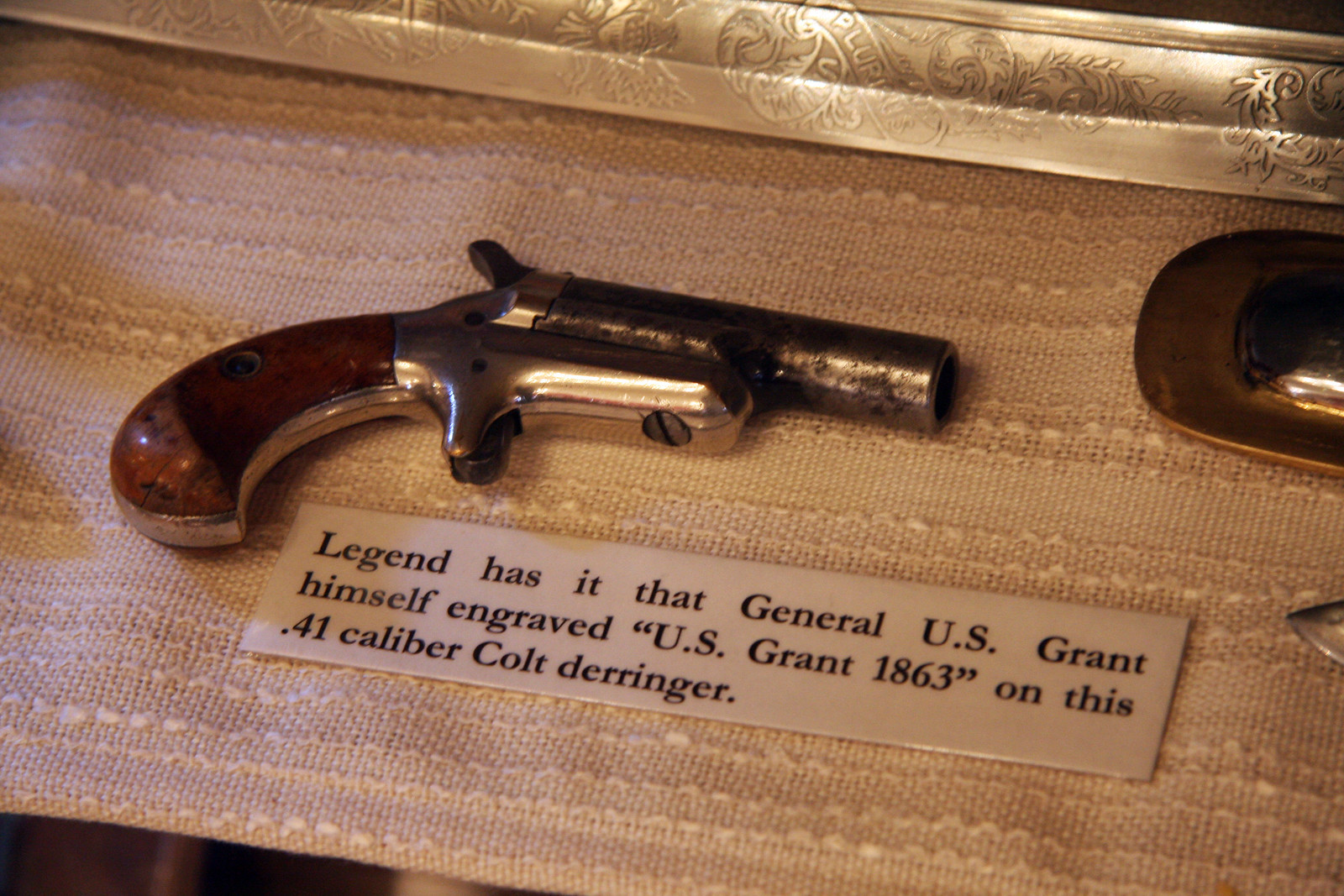This photograph captures a small, handheld Colt Derringer pistol displayed on a cream-colored cloth surface. The pistol, which is metallic silver with a brown wooden handle, has signs of corrosion, particularly around the barrel, which points to the right. A white, rectangular card beneath the gun provides historical context, reading: "Legend has it that General U.S. Grant himself engraved U.S. Grant, 1863, on this .41 caliber Colt Derringer." The gun appears to be on display, likely in a museum, emphasizing its historical significance. In the background, there's some vaguely visible embroidery or decorative elements, possibly resembling wreaths, adding to the presentation's ornate appearance. Additionally, another metal object can be seen near the right edge of the frame, contributing to the curated setting of the display.